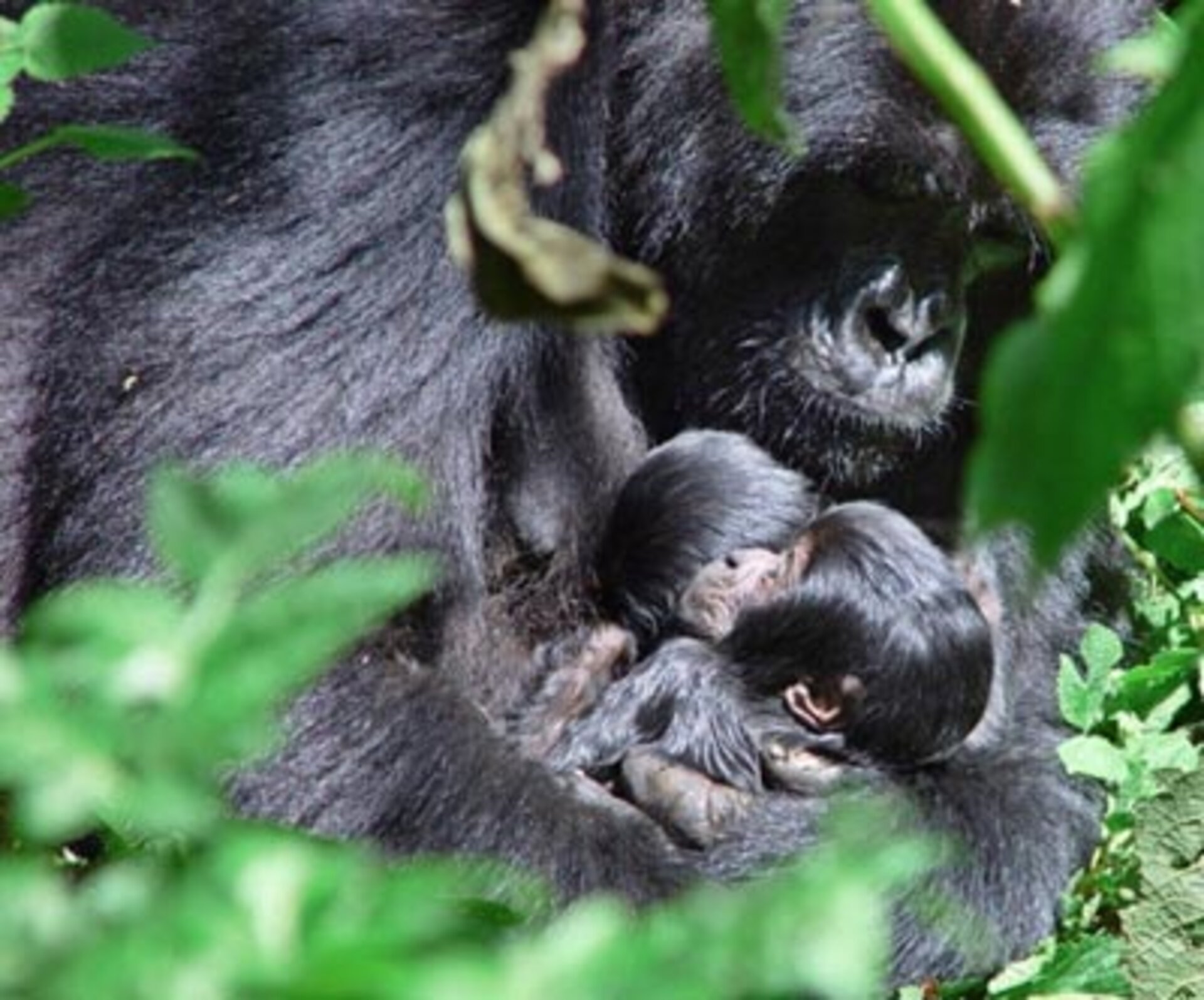This professional photograph features a close-up scene of a mother gorilla with her two baby gorillas, set against the backdrop of a lush, outdoor environment. The mother's black fur and dark facial skin contrast with the lighter skin of one of the baby gorillas, whose face is visible in profile. The mother is holding the two babies tightly in her arms, creating a protective and nurturing tableau. Leaves and plants in the foreground, vibrant green and slightly blurred, partially frame the mother, emphasizing her presence. The image captures the gorillas in sharp focus, highlighting their tender interaction amidst the natural, green surroundings.